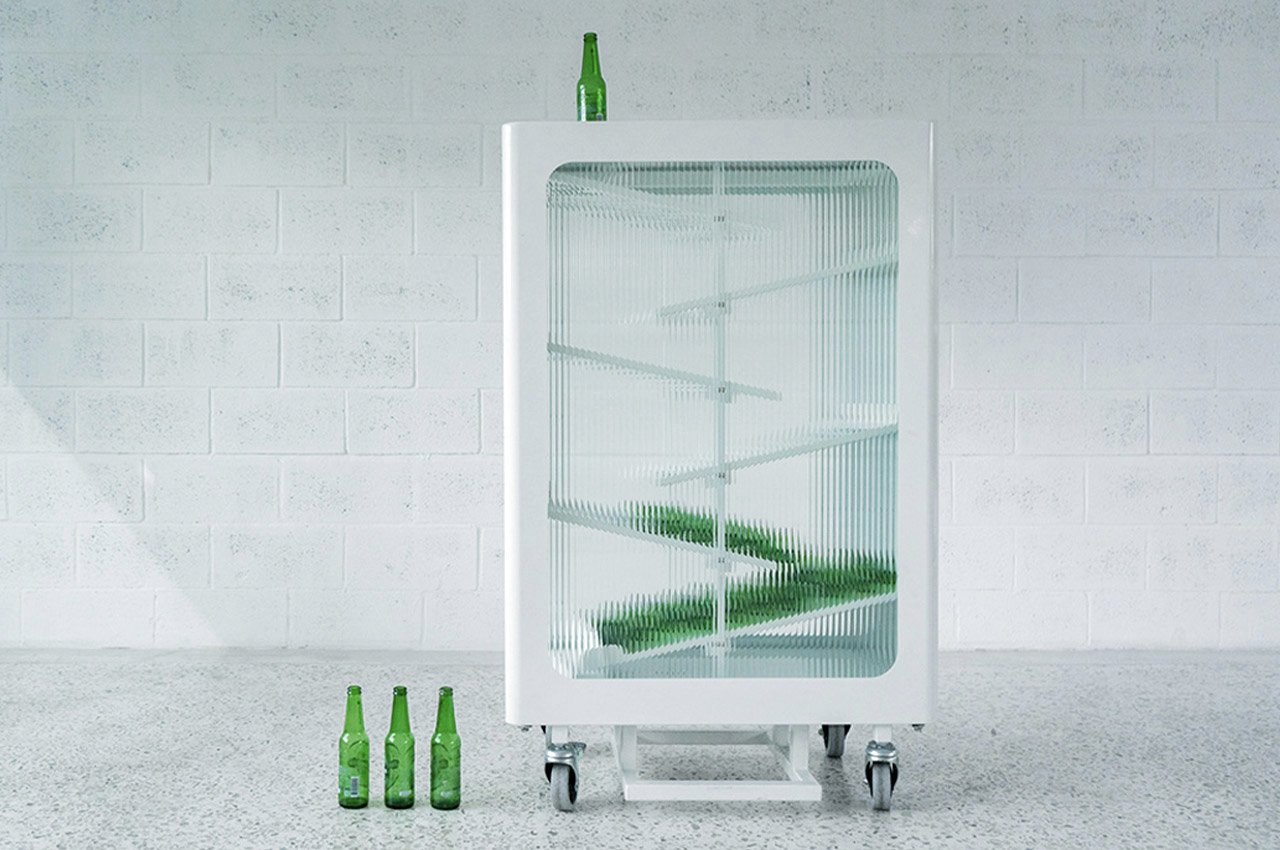In this landscape-oriented photo, set against a white brick wall, a distinctive container takes center stage. The container is rectangular, featuring a white exterior and supported by four wheels. The front surface is opaque with diagonal white shelves inside, vaguely visible, holding indistinguishable green items. The floor beneath is white with black speckles, resembling an epoxied surface. Atop the container, on the upper left corner, rests a single green glass bottle, likely a Heineken. To its left, close to the container's left front wheel, three additional green glass bottles are positioned on the floor. No people or text appear in the scene, with the primary focus being the container and the green bottles.